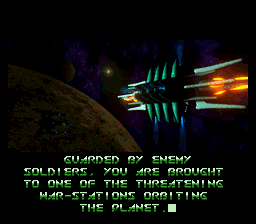In this captivating image set in the vastness of space, the viewer's attention is initially drawn to the lower portion, where text in a greenish gradient boldly declares: "GUARDED BY ENEMY SOLDIERS YOU ARE BROUGHT TO ONE OF THE THREATENING MAR STATIONS ORBITING THE PLANET," punctuated ominously by a green cursor mark. Dominating the background, a dark gray planet with rust-colored splotches looms, casting an eerie presence over the scene. To the middle right, a futuristic craft—possibly a satellite or a spaceship—floats, characterized by a central round portion flanked by wing-like extensions on each side. This vessel features intricate green light outlines and orangish-lit sections on its wings, with additional blue lights accentuating the middle. Further in the distance, another celestial body appears as a subtle silhouette against the backdrop of space, accompanied by the faint glimmer of a distant star. Adding to the complexity of the scene, a vague object with bluish lights—potentially another satellite or ship—hovers in the background, contributing to the overall sense of mystery and tension.